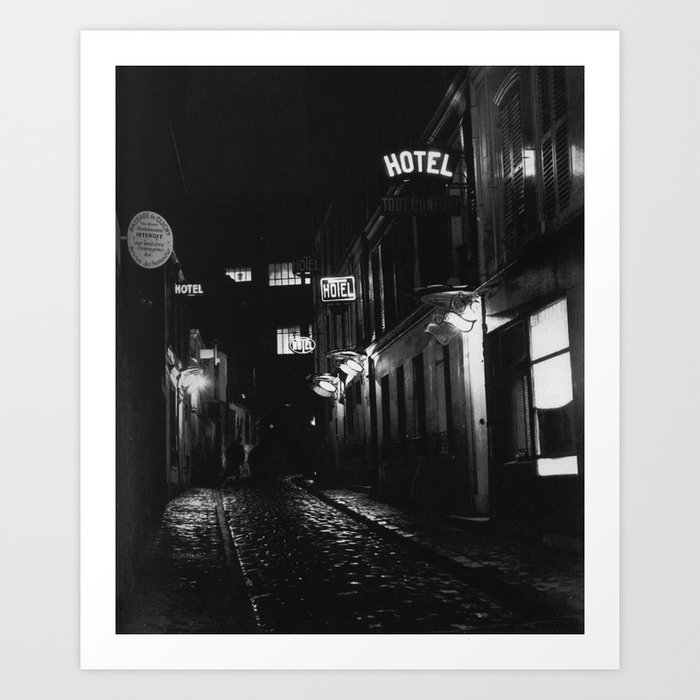This image is a black and white photograph with a white border, approximately a quarter to a half inch wide, situated against a light gray background. The overall dimensions of the image are about five inches high and five inches wide, with the photo itself being around four inches high and three inches wide. The photograph captures a narrow, cobblestone-paved street at night, flanked by small sidewalks on both sides. Tall buildings line the street, their windows illuminated by lights, casting a glow on the scene below. 

Neon hotel signs are prominently displayed, three on the right side and one on the left, with additional signage in the background, including a circular sign that reads "passage to Clichy." One of the hotel signs on the right is not illuminated. The vintage look of the hotel signs suggests a 1930s or 1940s style, adding a historical ambiance to the alleyway. Above the buildings, more signs protrude into the night sky, creating a dense, atmospheric urban scene reminiscent of old city streets.